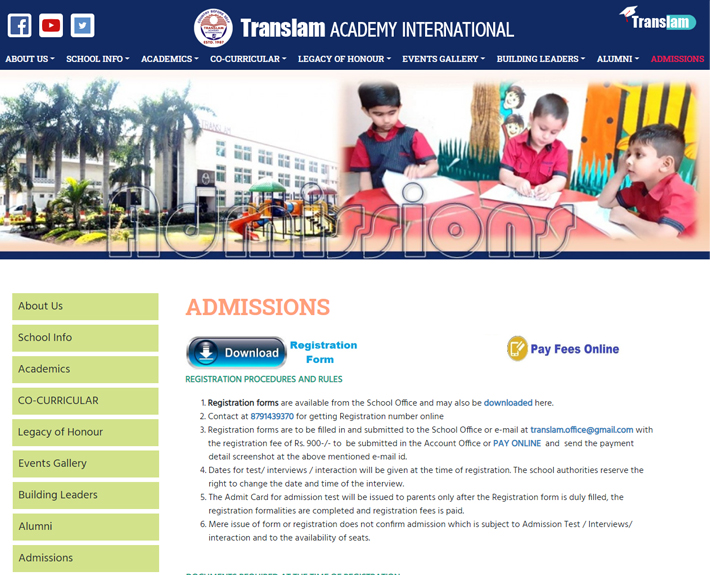The image is a screenshot of a web page for Trans-Lamb Academy International. At the center of a dark blue horizontal banner, the site's name, "Trans-Lamb Academy International," is prominently displayed in bold white text. In the upper left corner, icons for Facebook, YouTube, and Twitter are visible. In the top right, the word "Trans-Lamb" appears in white with a horizontal navigation menu underneath. This menu lists options in white text with downward-facing arrows next to each: About Us, School Info, Academics, Co-Curricular, Legacy of Honor, Events Gallery, Building Leaders, Alumni, and a red-highlighted Admissions at the end.

Below the banner, there is a broad horizontal image featuring a row of palm trees in front of a large, three-story industrial-looking white building. On the right side of this image, three preschool-aged boys wearing matching red shirts with black-trimmed sleeves are sitting at an orange school table, engaged in some paper activities.

Centered below this image, "Admissions" is prominently displayed in red at the top left. Beneath it, a blue button labeled "Download" with a white down arrow is located, followed by the text "Registration Form" in blue to the right. To the far right, the phrase "Pay Fees Online" is in dark blue next to a tan icon. Below this, "Registration Procedures and Rules" is highlighted in green, with six numbered lines detailing registration procedures.

On the far left, a vertical column of green rectangles presents a menu with black lettering listing: About Us, School Info, Academics, Co-Curricular, Legacy of Honor, Events Gallery, Building Leaders, Alumni, and Admissions.